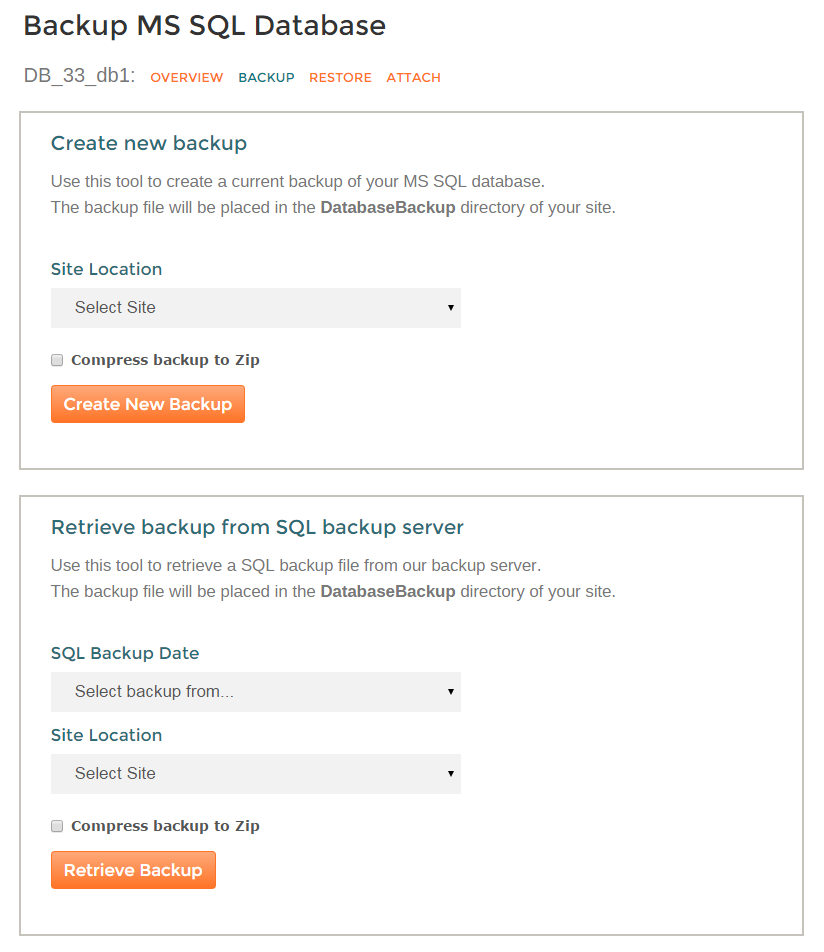The screen display shows an interface for managing MSSQL database backups. At the very top, there is a heading titled "Backup MSSQL Database - db__33__db1 Overview." The interface includes several sections surrounded by bordered lines.

1. **Create New Backup**:
   - Tooltip/Instruction: "Use this tool to create the current backup of your MSSQL database."
   - Action Button: "Create New Backup."
   - Process Info: "The backup file will be placed in the database backup directory of your site."
   - Additional Elements: A dropdown menu allowing the user to select the site location for the backup. Users are guided to ensure the backup file is compressed into a zip format.

2. **Retrieve Backup**:
   - Tooltip/Instruction: "Use this tool to retrieve the MSSQL backup file from our backup server."
   - Action Button: "Retrieve Backup."
   - Process Info: "The backup file will be placed in the database backup directory of your site."
   - Backup Date: An option to select the backup date from a dropdown menu, ensuring the correct backup is retrieved.
   - Additional Elements: Instructions similar to those in the creation section regarding the verification and placement of the backup zip file.

The entire section is designed with user-friendly tips and clearly marked actions to streamline the process of creating and retrieving MSSQL database backups. The layout is organized with bordered lines, ensuring each tool's function is easily distinguishable.